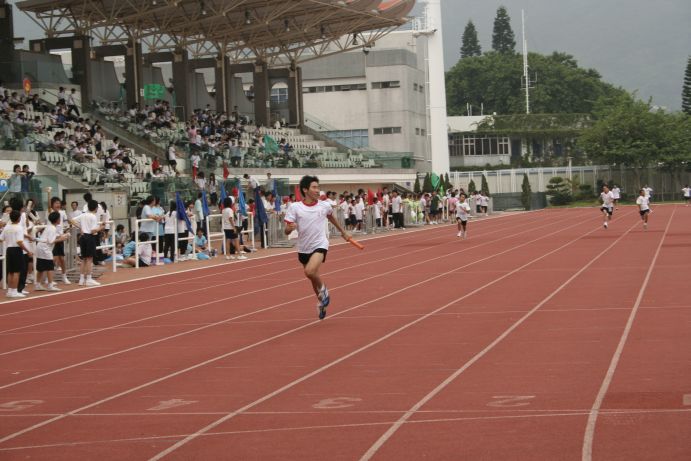The color photograph captures a lively track race taking place on a large outdoor racetrack. The image prominently features lane numbers 1 through 9, with the cameraman positioned in front of lane 2. Dominating the scene is an Asian male, dressed in a white t-shirt and short black shorts, running far ahead of his competitors in lane 4. He is holding an orange baton, signifying that this is part of a relay race. The runner looks over his left shoulder to check the position of the trailing racers, who are quite far behind, with three notably distant yet visible. The stands on the top left-hand corner of the photo are filled about halfway to two-thirds with spectators, while people dressed in uniforms, likely other competitors or team members, are seen on the sidelines clapping and cheering. In the far background, lush green trees and a small modern-looking white house with a surrounding fence complete the setting. The overall impression suggests the event possibly taking place in an Asian country, indicated by the ethnicity of the runners and the design of the surroundings.